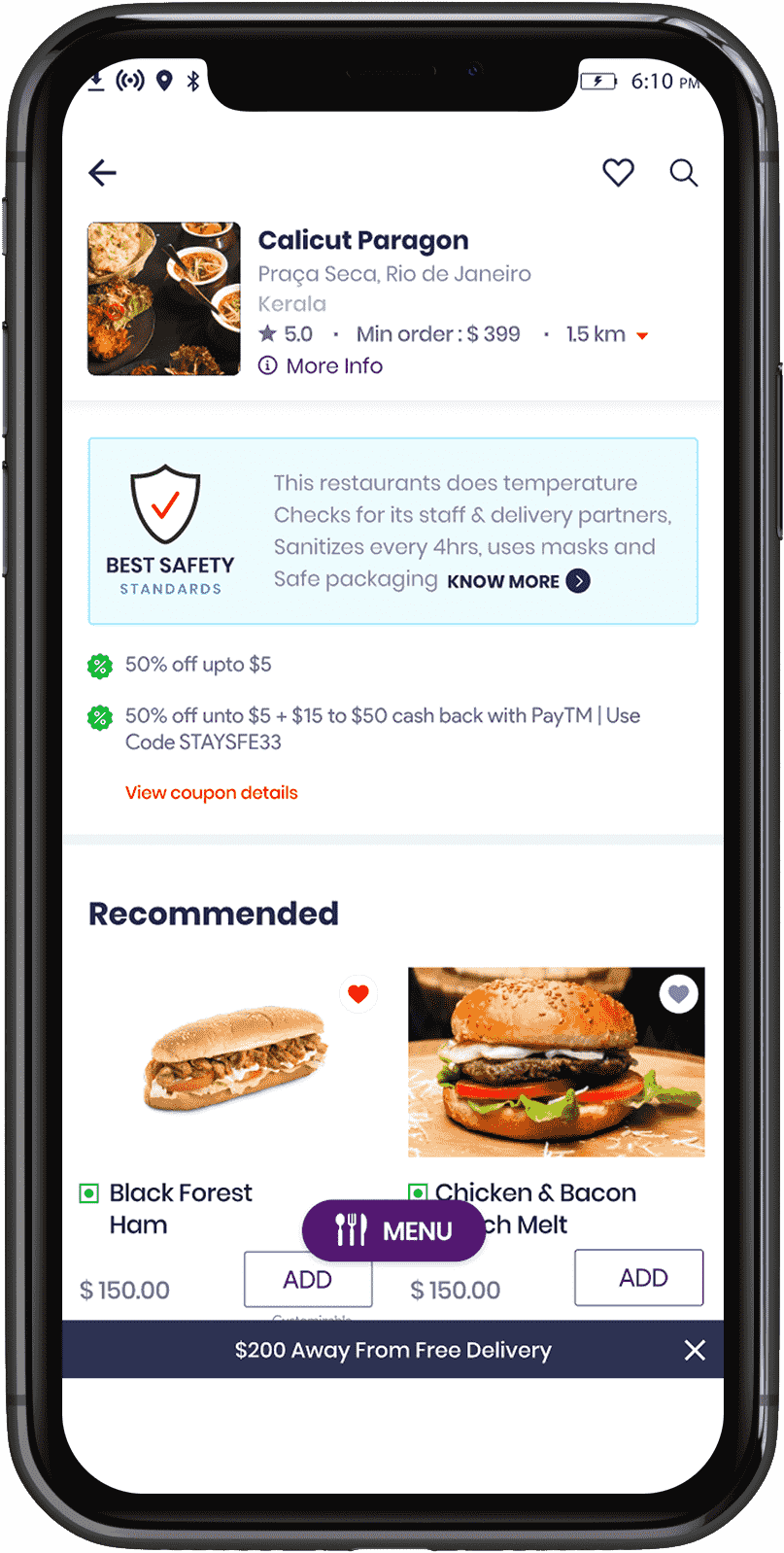This image features an app displayed on a black smartphone. The screen shows a white background with the interface of a restaurant listing. At the top, there is a back button on the left and a heart icon and search button on the right. Below these icons, the restaurant name "Calicut Paragon" is displayed, alongside its location in Praca Seca, Rio de Janeiro, Kerala, and a perfect rating of 5.0 stars. The minimum order value is $399, and the restaurant is 1.5 kilometers away. 

There is a tab labeled "More Info," and the text beneath highlights the restaurant's adherence to top safety standards, mentioning regular temperature checks for staff and delivery partners, sanitizing every four hours, mask usage, and safe packaging. A clickable option invites users to see more details.

Further down, there's information about limited-time offers, including a 50% discount up to $5, a cashback offer between $15 to $50 when using PayTM with the code "StaySafe33," and a link to view coupon details. 

The image also showcases sandwich recommendations, specifically a "Black Forest Ham" sandwich and a "Chicken and Bacon Lunch Melt."